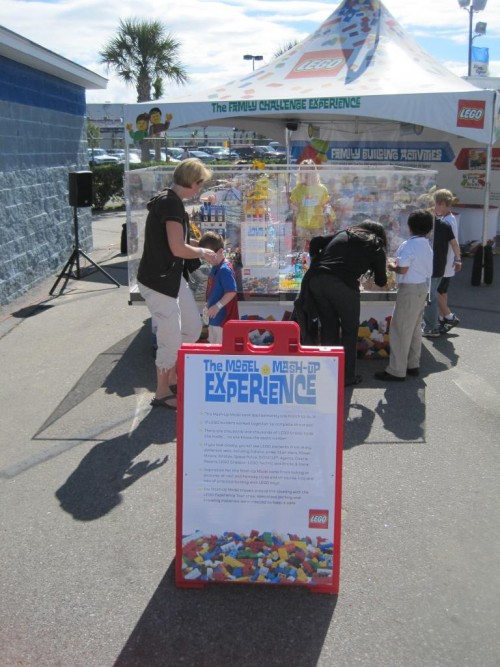In the foreground of the photograph, there is a prominent red sign sitting on the ground, featuring the words "The Model Mashup Experience" in a mix of large and small, capital and lowercase blue text. Beneath this title, in smaller black text, are six lines of text too tiny to read from this distance. At the bottom of the sign, there's an image of a huge stack of Lego blocks and slightly to the right sits the iconic Lego logo.

Behind the sign stands a kiosk resembling a large aquarium with high, see-through glass walls filled with various Lego models and items. The glass container sits atop a table and is open from the top. Around this setup, a mixture of adults and children are gathered, some appearing to engage with or observe the display. In particular, there are two women with their young boys standing in front of the kiosk. 

The kiosk itself is shaded by a white umbrella or canopy, prominently displaying the red Lego logo on the right-hand corner. On the left-hand corner of the canopy, two Lego characters are visible, and the words "The Family Challenge Experience" are inscribed in the middle. This scene is set against the backdrop of what appears to be a parking lot next to a shopping mall, with cars and buildings visible in the distance along with a tree and a speaker on a stand nearby.